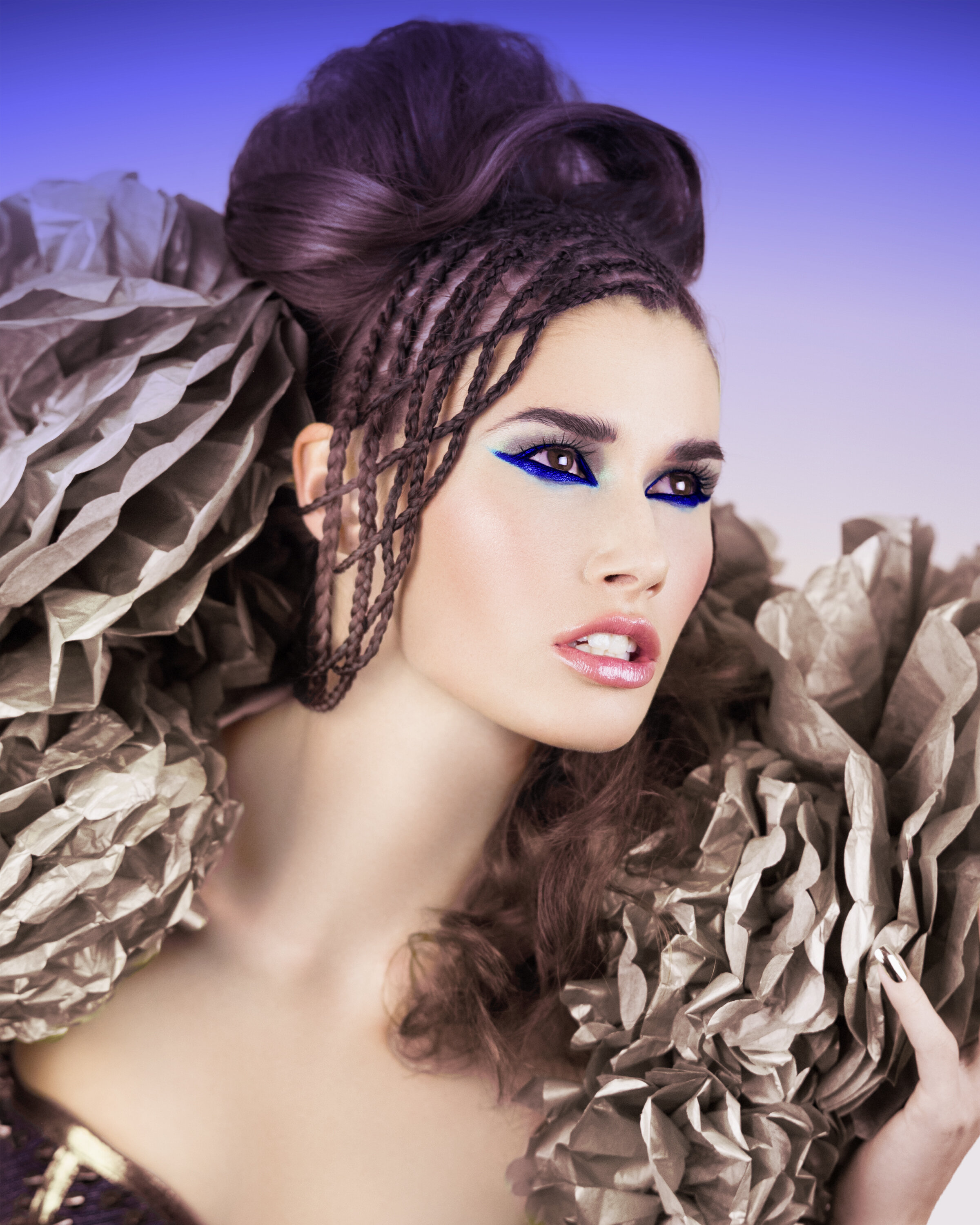This photograph, potentially a realistic AI rendition, captures a detailed portrait of a Caucasian woman with light skin and dark brown eyes. Her dark brown hair is styled intricately; the front section is composed of thin, long braids cascading over the right side of her face, while the back portion is voluminous and pinned up, forming a big puff. Her makeup is striking, featuring dark blue graphic liner, heavy mascara, and a combination of dark and light white eyeshadow. Her arched eyebrows are meticulously shaped, and she wears bright pink blush, highlighter, and pink lip gloss. Her teeth are visible in a slightly clenched, open-mouth expression.

The woman's attire is reminiscent of a Spanish dancer's costume with a touch of Mardi Gras flair. She is dressed in a shiny, possibly sequined gown, which includes gold and brown elements. Notably, her dress has elaborate golden ruffles on the left side, extending almost to the top of her head, and similar puffy, ornamental shoulders. One visible finger is adorned with metallic silver nail polish. The background gradates from a dark blue to a lighter shade towards the center, enhancing the dramatic effect of her appearance.